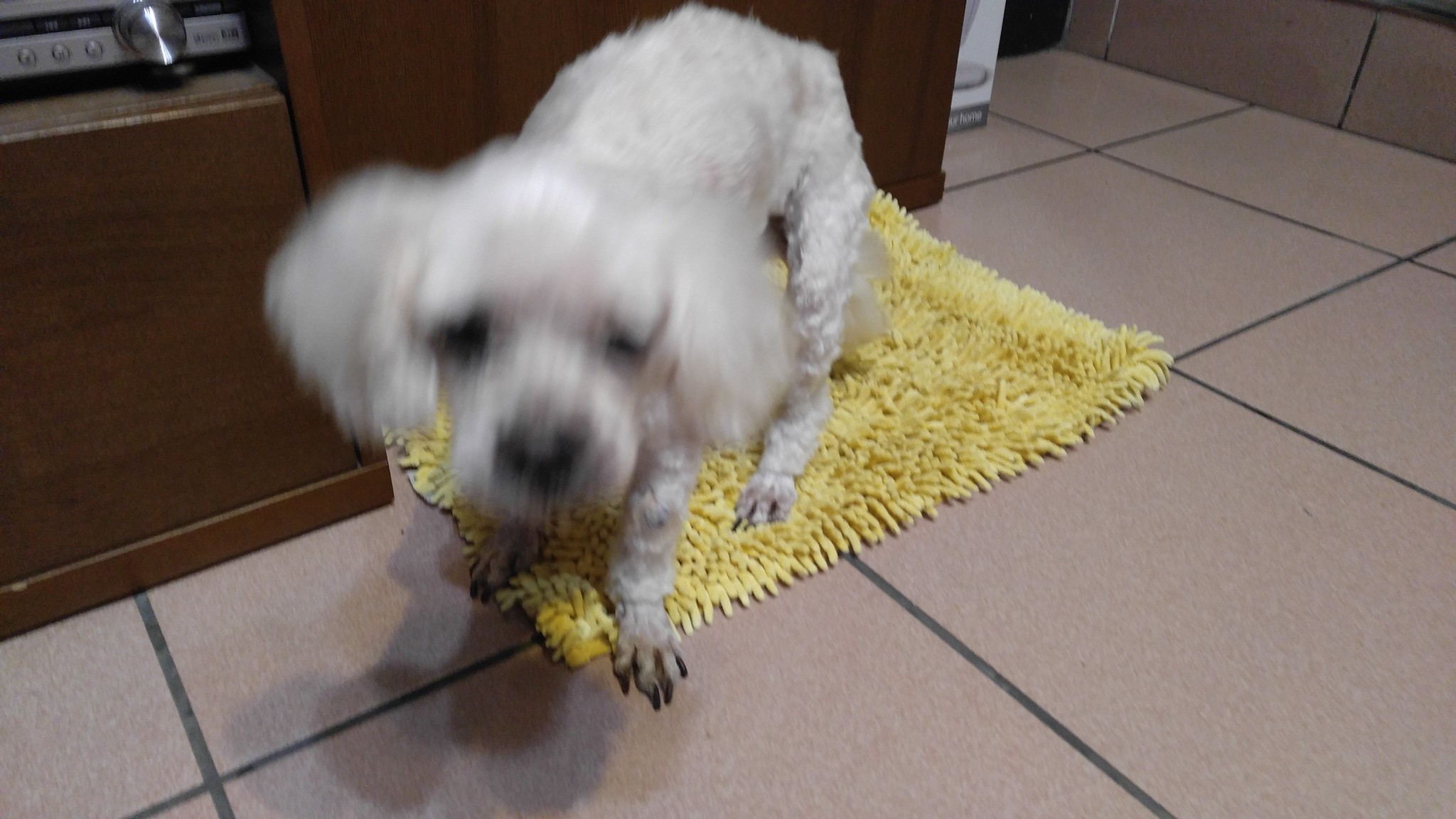In this blurry, horizontal photograph, a frail-looking, older white poodle stands on a yellow chenille bathroom rug. The poodle's face is particularly out of focus, creating a double-exposure effect. Its black eyes and long nails add to its delicate appearance, while its posture seems weak or hunched. The scene is set in front of a medium-brown stereo cabinet that appears somewhat inexpensive. Part of a tuner is visible in the upper left-hand corner of the image. The rug beneath the poodle lays on a beige tiled floor, comprised of larger tiles interspersed with gray grout.